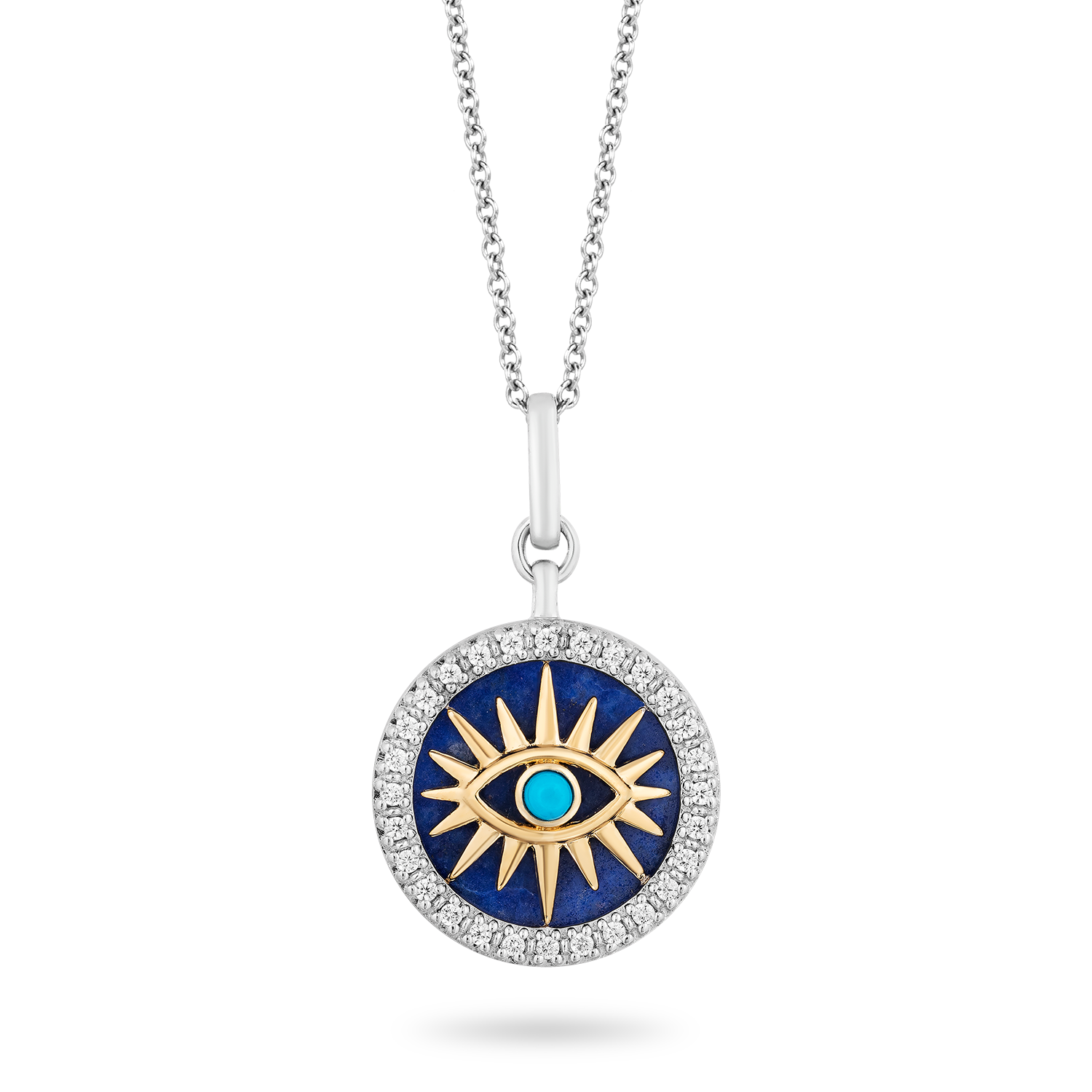This detailed digital illustration showcases a silver necklace pendant hanging from a medium-link silver chain. The pendant, predominantly round, features a dark blue circular background with an intricate design. Central to the pendant's motif is a golden eye, with a turquoise pupil and encircled by golden sun rays. Flanking the outer edge of the pendant are numerous diamond-like gemstones, adding an elegant sparkle. The pendant casts a light gray shadow, enhancing its dimensional presence in the image. The predominant colors throughout this close-up screenshot include silver, blue, gold, and light blue, capturing the ornate beauty and intricate details of the jewelry piece.